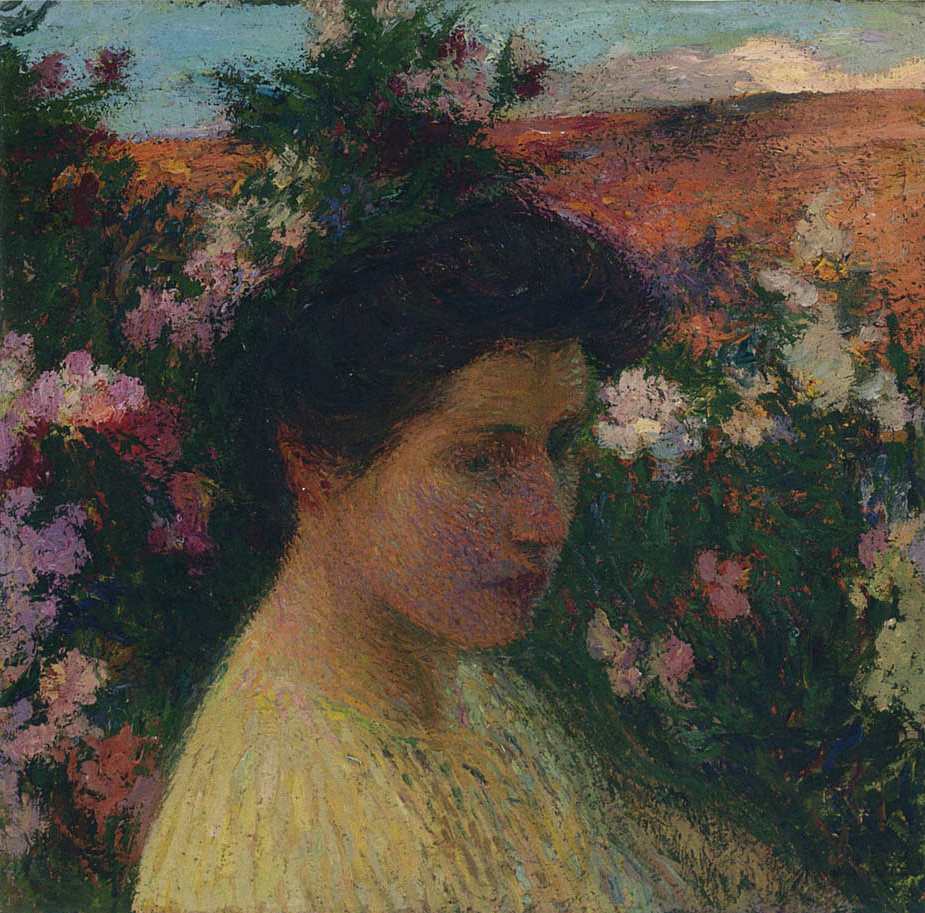The painting is a square, Impressionist oil artwork from around the 1900s. It prominently features a woman with dark hair styled in a thick bob, wrapped behind her head. Her complexion is whitish with hints of bluish tones on her cheeks, and she appears to be gazing slightly to the bottom right. The woman is adorned in a light-colored, stringy yellow dress embellished with subtle, yet colorful gems in purple, blue, and green tones. The dress and the woman's figure are depicted with rough, vertical brush strokes characteristic of Impressionist technique.

In the background, a serene landscape unfolds with a blue sky and scattered white clouds along the horizon. Below this sky, a stretch of brown and red-toned earth or hilly terrain creates a grounding effect. Surrounding the seated woman, there is a lush abundance of green shrubbery and a vibrant array of flowers. To her right, colorful blooms in white and pink populate the scene, while on her left, the floral display extends upwards, integrating white, pink, and red flowers, possibly mingling with bushes or trees. The entire composition adopts a speckled and streaked approach in line with the traditional Impressionist style, culminating in a vivid and evocative portrayal.